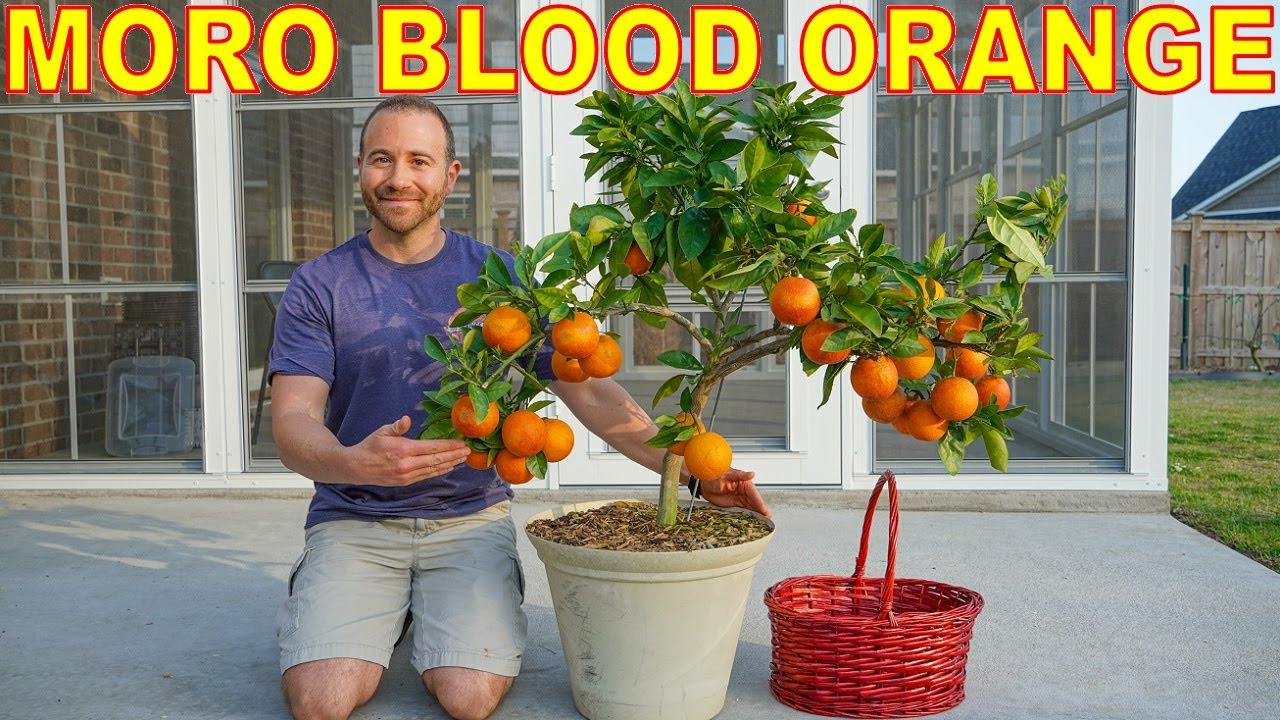The image is an outdoor advertisement for Moro Blood Orange, featuring a lively, bright daytime setting. At the top of the rectangular image, the words "MORO BLOOD ORANGE" are prominently displayed in bold, all-caps yellow letters outlined in red. Below, a man with a beard, dressed in a blue heather t-shirt and tan khaki shorts that fall just above his knees, is kneeling on a concrete patio. He's positioned towards the left side of the image, smiling with his right arm bent in front of his stomach. Beside him, and reaching to the top of his head, is a flourishing orange tree in a tan pot, laden with vibrant, bright oranges. Just to the right of the tree sits an empty red wicker basket. In the background, there is a glass-enclosed sunroom attached to a red brick house, supplemented by a fence and patches of grass, all clearly lit by ample natural sunlight.